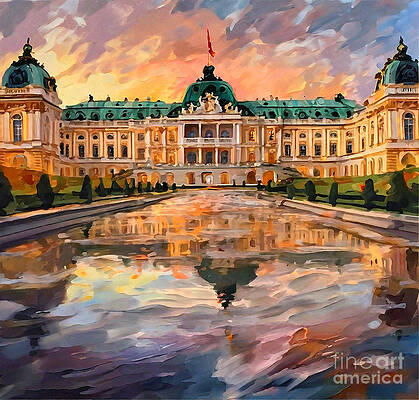This painting, possibly rendered in oil or acrylic, captures a grand mansion or castle distinguished by its expansive layout and architectural flair. The large, rectangular building is accentuated by its multiple towers and wings, giving a monumental feel reminiscent of a government building or a museum. Its walls are painted in shades of yellow and cream, adorned with gold accents, while the roof and central dome are a distinctive green. The mansion stands fronted by a wide, man-made reflecting pool, capturing the vivid colors of the sky—hues of yellow, pink, purple, and blue—mirroring them beautifully in the water below. Framed by meticulously trimmed hedges on either side, the estate's grounds showcase lush greens and carefully shaped botanical art. The scene, viewed from an approach perspective, is visually anchored by the vibrant sky contrasting harmoniously with the estate's stately architecture. The piece is signed "Fine Art America" in the lower right corner, and it vividly employs a palette that spans green, yellow, cream, orange, brown, and gold tones.